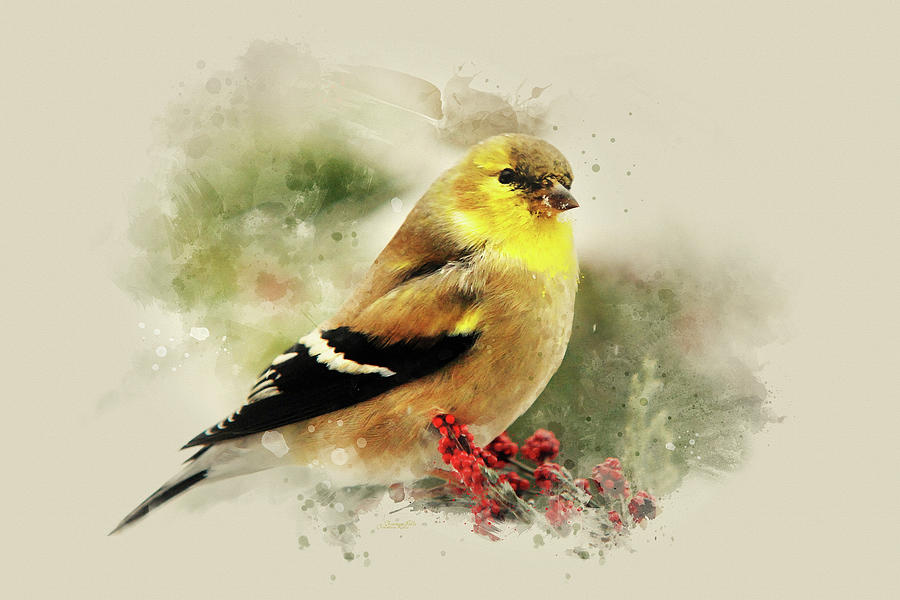This rectangular image, approximately six inches wide and four inches high, features a meticulous depiction of a yellow canary perched on a branch dotted with small red berries. Set against a background of light brown, tan, and green smudges, possibly suggesting foliage, the canary commands the foreground with impressive detail that borders on photorealism.

The bird faces right, showcasing its vibrant yellow neck and chest. Its head sports a small light brown dome that seamlessly blends into the brilliant yellow around its eye. The black, circular eye and the small, pointed beak—brownish-black at the tip and lightening to gold near the face—add to the canary's lifelike appearance.

Further down, the bird's body reveals a blend of light brown and yellow streaks extending to the upper part of its wings. The tips of the wings are black with a crisp white stripe in between, contributing to the detailed texture of the feathers. The bird’s belly transitions from a light brown to a whitish hue, and its tail continues this pattern with subtle black markings.

The overall composition combines elements of watercolor artistry and possibly mixed media, with the canary’s detailed rendering suggesting a contrast to the more abstract, smudged background.